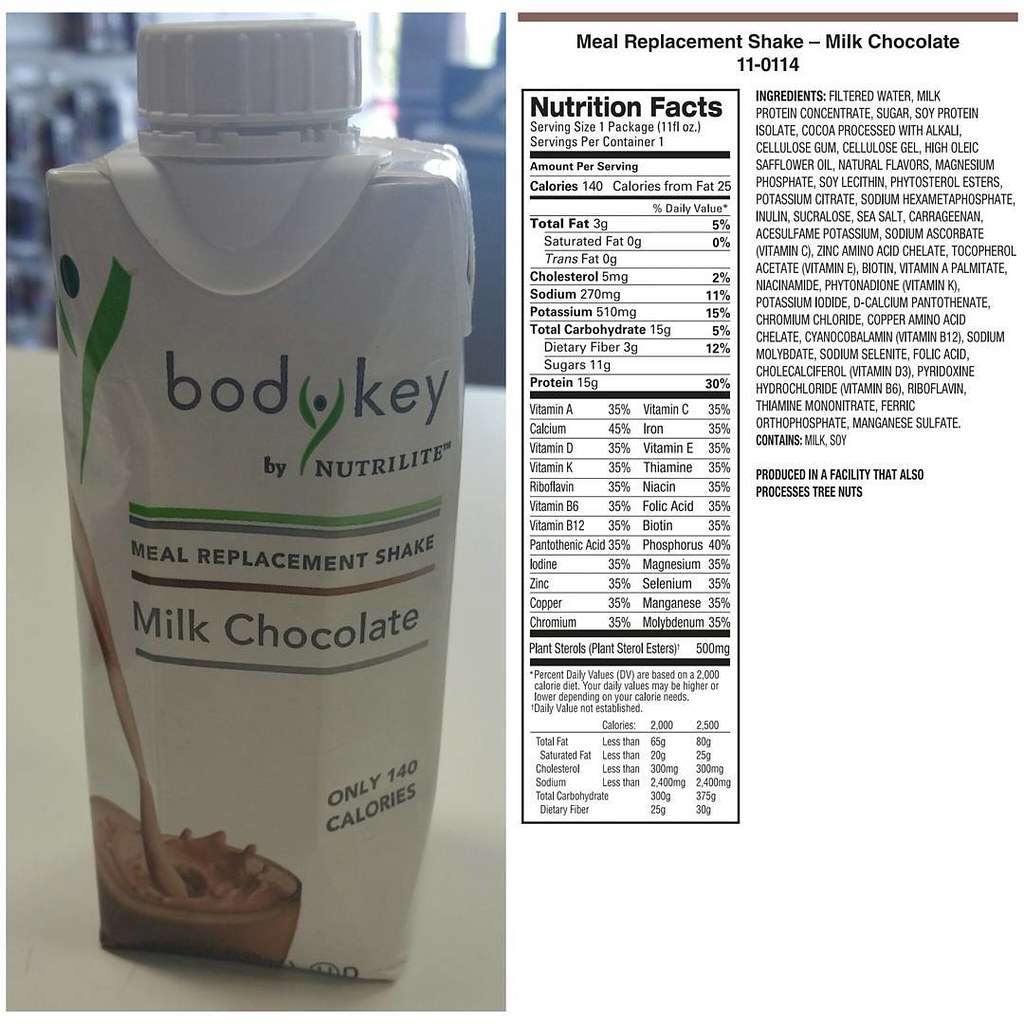The photograph showcases a meal replacement shake in a distinctively shaped white bottle with a white screw-on cap. The label boldly features the brand name "Body Key" by Nutrilite, with "BOD" in dark blue and an artistic representation of the letter "Y" formed by two dark blue leaf-like shapes with a dot in the center. The word "Key" appears in a gradient transitioning from blue to dark blue. Below this, a green line is followed by the text "meal replacement shake" in dark blue, along with "milk chocolate" on a brown line and a gray line beneath it.

An image of milk chocolate being poured into a clear glass is prominently displayed on the label, with a rich dark brown liquid splashing within the glass. To the right of the bottle, the label highlights "only 140 calories" in dark blue text. Adjacent to the bottle is a detailed nutritional facts graphic, listing essential information such as calories, total fat, cholesterol, sodium, potassium, total carbohydrates, protein, and a comprehensive list of ingredients. The bottle's shape is notably non-circular, described as almost hexagonal with a slightly textured feel, designed possibly for better grip.